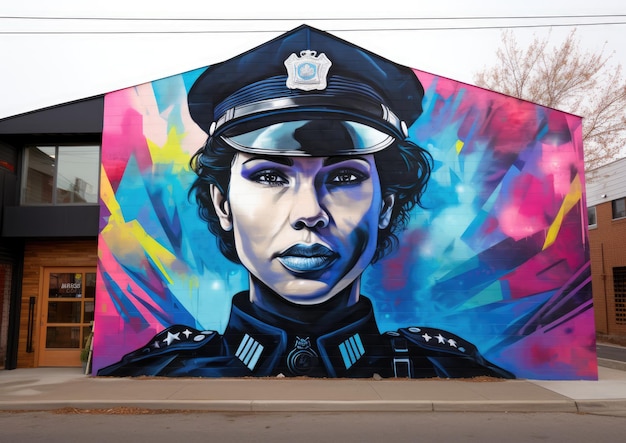This photograph, taken on a clear, sunny day on a residential street, captures an expansive and vividly colorful mural painted on the front of a two-story building with a peaked roof. The building’s original black exterior frames the mural, which prominently features a stoic female police officer from the neck up. Her face, painted in a style reminiscent of the Obama Hope posters, exhibits light blue lips, gray skin with blue accents along her cheekbones, and purple around her eyes, contrasted by her gray-colored eyes. She wears a dark blue police hat adorned with a gold badge and a black brim that reflects white and purple hues. Strands of black and blue hair peek out from beneath her hat, draping over her ears. Her uniform is black with a blue collar, decorated with four lines on each side and epaulets bearing stars and buttons on her shoulders. The mural’s background bursts with dynamic colors, including bright blues, pinks, yellows, and purples. To the left of the mural, a brown-framed window and a wooden door frame punctuate the black facade of the building. The sky in the background appears hazy, and two power lines stretch horizontally across the scene. Nestled to the right of the building is a tree with bare branches. No text is present within the image, making the mural the central focus of this striking and detailed composition.